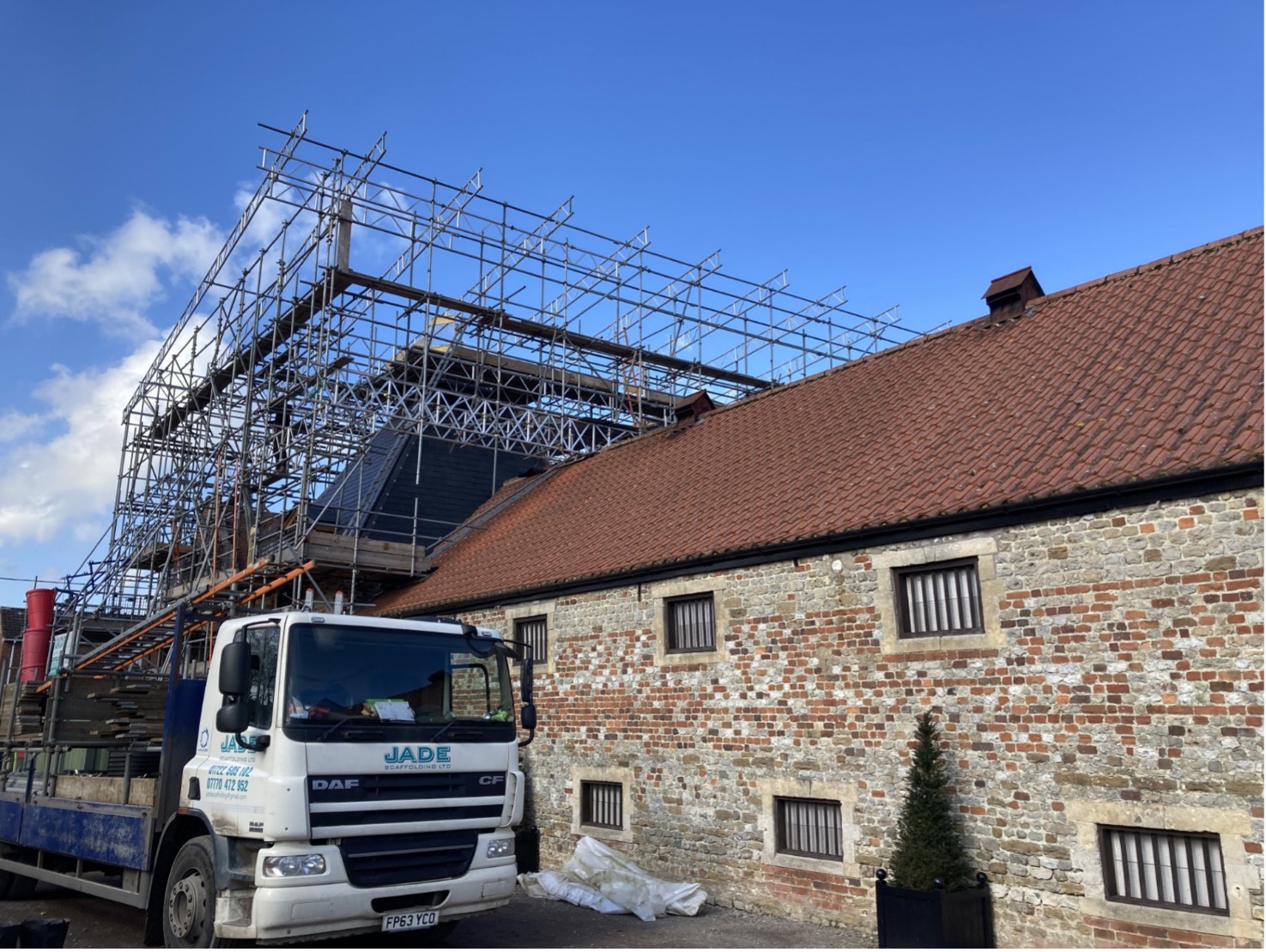This color photo depicts an ongoing construction or restoration project on an older, whitewashed brick building with a prominently worn exterior. The building, possibly located in the UK given its architectural style, features a pitched tile roof and is flanked by six barred windows, three on the upper level and three on the lower level, evoking a sense of an old warehouse. The right side of the frame shows extensive scaffolding surrounding the end of the building and extending to a higher gray roof, indicating active construction work possibly aimed at expanding or reinforcing the structure. 

A vibrant blue sky with scattered clouds enhances the setting, while a triangular-shaped potted tree adds a touch of greenery beside the building. At the forefront of the image, a white flatbed construction truck marked "Jade Scaffolding Limited" is parked, bearing a license plate that reads FP63YCO. The truck, equipped with a ladder, suggests engagement in the construction work. White bags of materials are scattered on the ground in front, further emphasizing the ongoing nature of the project. The overall scene blends historical architecture with modern construction, reflecting an intersection of preservation and progress.